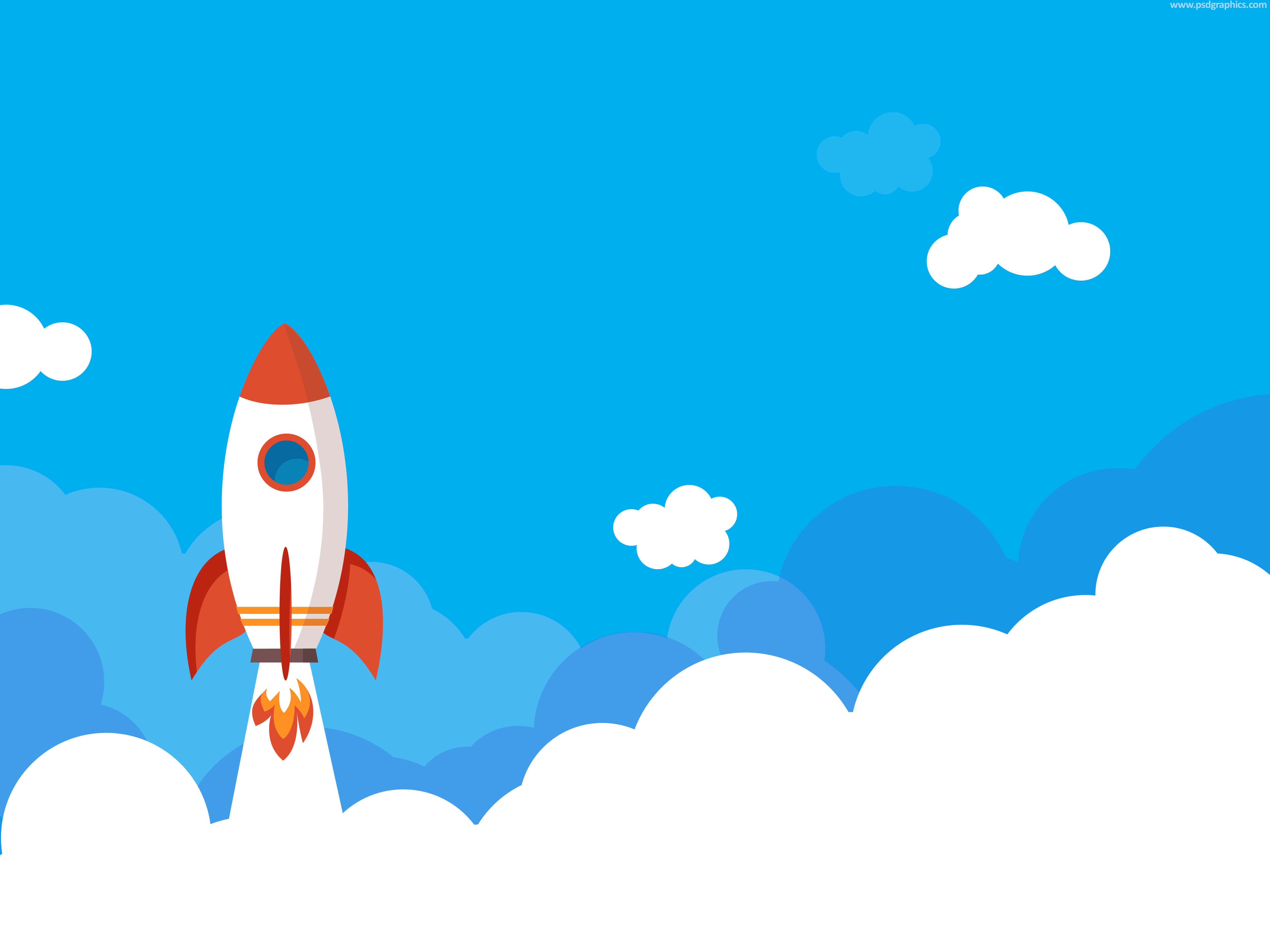The image is a highly detailed, computer-generated cartoon of a small rocket ship blasting off into a light blue sky. The rocket, positioned to the left of the center, is predominantly white with an orange stripe around its body. It features a distinct red nose cone and has two orange, shark fin-shaped wings with red stripes. A blue bubble-shaped window, outlined in red, is situated on the rocket's side. Beneath the rocket, an orange flame and white smoke trail mark its ascent. 

The sky is a varied shade of light blue, filled with four puffy clouds—three bright white and one faint light blue that almost blends into the sky. The bottom of the image fades into white, enhancing the impression of elevation and distance. The image is notable for its clean, polished, and highly stylized aesthetic, indicative of high-quality digital artwork. There are no other elements such as text, numbers, people, or animals in the scene, focusing purely on the rocket's journey upward.